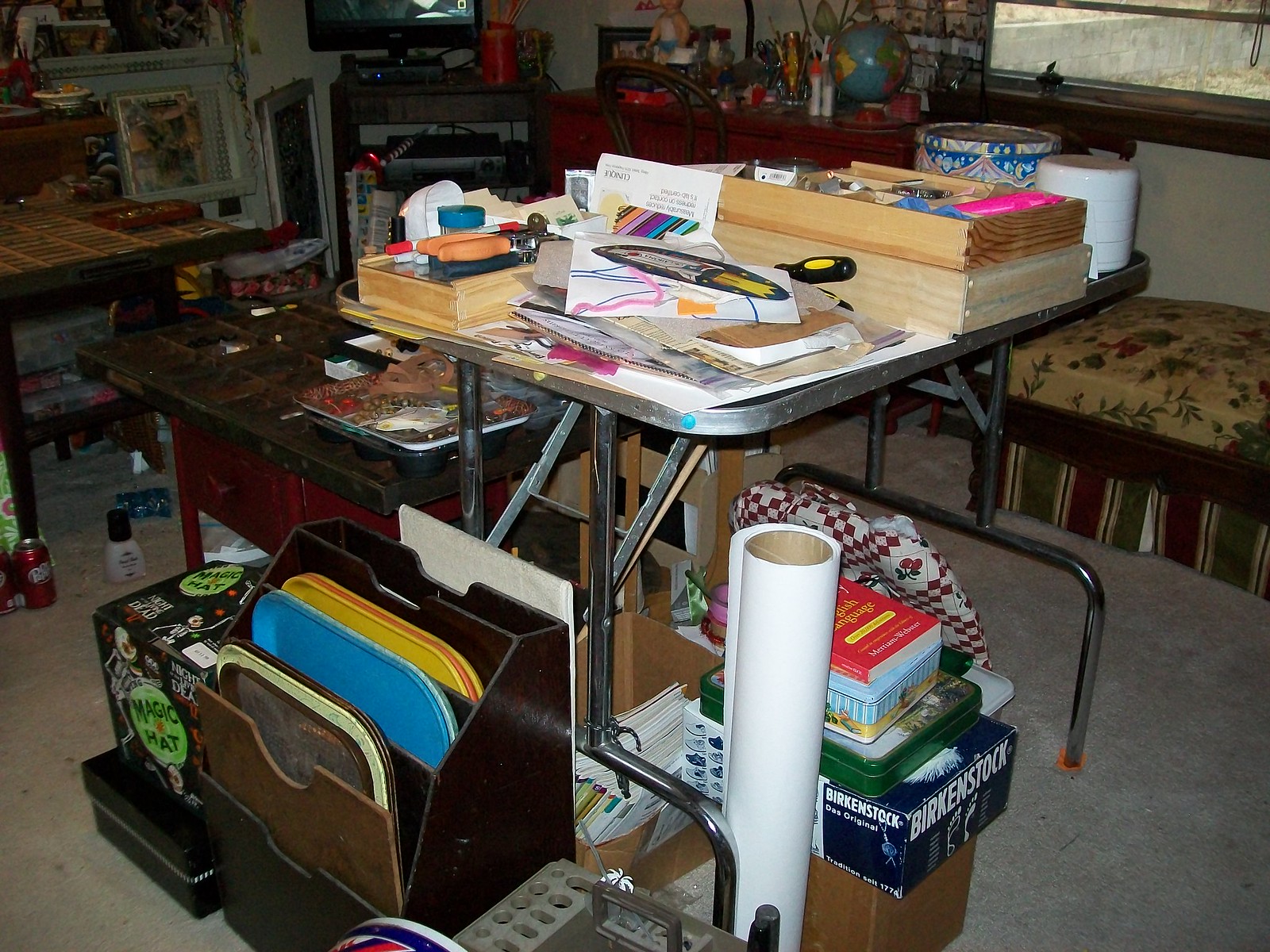The image depicts the cluttered interior of a design space, characterized by a gray carpet that covers the floor. In the distant background, a countertop is adorned with an assortment of knickknacks, notable among them a blue globe with yellow landmasses. Various bottles and containers of different shapes and sizes are scattered around, one of which holds pencils and fizzy sticks. A small figure wearing a white shirt, blue pants, and having yellow skin — seemingly a toy or figurine — stands in the far background.

An open window in the top right corner reveals an exterior view of a stone wall and some green grass. Nearby, a container predominantly blue with yellow and red stripes, and a white jar can be seen. Below them, there is an ornament, possibly a footrest, covered with yellow fabric. 

Towards the bottom of the image lies a large white tube, alongside which rests a red book with yellow text. Several metallic containers are placed nearby, including a blue and a green one, as well as another blue container labeled "Birkenstock." 

A cluttered table tops the scene, laden with an assortment of papers, knickknacks, and various brown rectangles. There is also a noticeable stack of what appears to be brown rolls or handles and a colorful piece of paper. To the left sits a file organizer with trays in white, blue, and yellow hues. 

Next to the organizer, a box marked with a green circle and black text reading "magic hat" can be found. Scattered on the carpet in the foreground are a makeup bottle and a video game controller. Above this cluttered scene, a tiled countertop is visible, reflecting the light from a TV or an entertainment system in the very bright background.